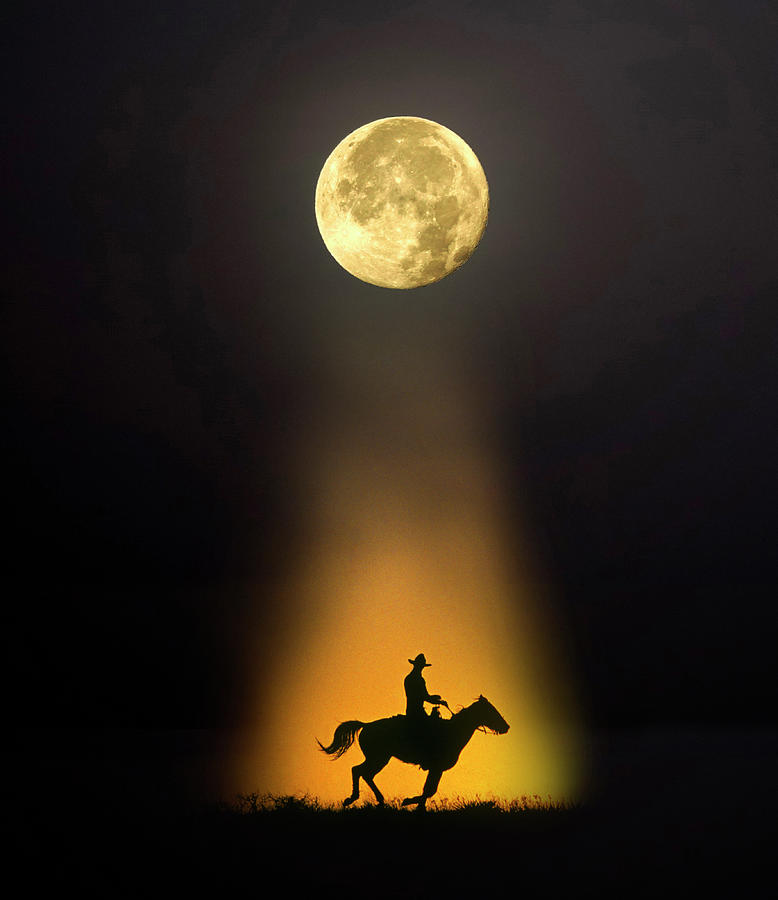In this art piece, a man on a horse is depicted as a silhouette or shadow, centrally positioned towards the bottom of a vertically-oriented rectangular image. He wears a cowboy hat and is illuminated by a yellowish-orange light. Above him, the full moon radiates the same yellow light, casting an ethereal glow that transcends downward, enhancing the dark, black background. The foreground features a grassy field, colored in shades of yellow and orange, blending into the light rays that bathe the rider. There is no text within this image, and the predominant colors are black, yellow, beige, and gray. The setting evokes a dreamy, celestial scene, seamlessly combining elements of night and light in a painting-like style.